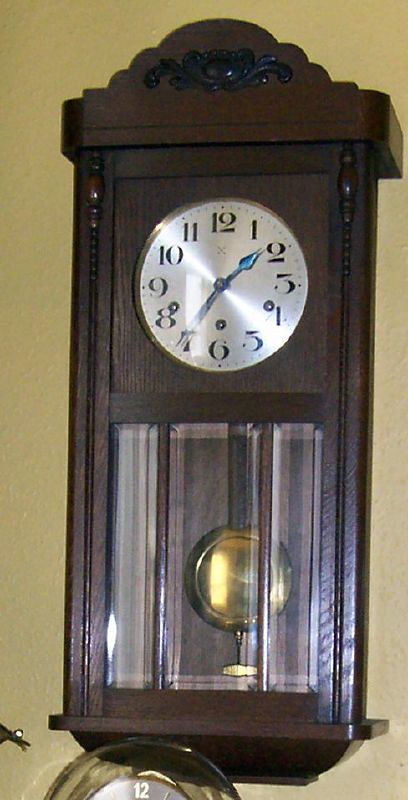This photograph showcases a striking clock mounted on a cream-colored plaster wall. The clock, constructed from richly stained dark wood, presents an elegant rectangular shape with a gracefully curved top. Its face, framed within the wooden structure, is adorned in a pale silver color, featuring clear black numerals. The hands of the clock are an eye-catching bright blue, adding a contemporary touch to its classic design. Below the clock face, a glass window reveals an intricate chime mechanism and a round pendulum suspended on a slender pole, enhancing the clock’s timeless charm.